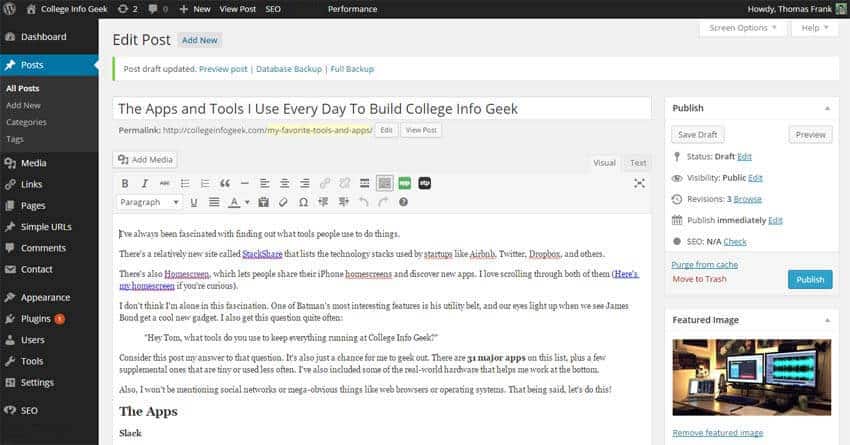This image showcases a detailed view of a website or web page titled 'College Info Geek.' In the top left corner, the site name and logo are prominently displayed. The interface includes an extensive sidebar menu with various tabs and drop-down options such as Dashboard, Posts (with sub-options for 'All Posts,' 'Add New,' 'Categories,' and 'Tags'), Media, Links, Pages, Simple URLs, Comments, Contact, Appearance, Plugins (highlighted with a red notification dot), Users, Tools, Settings, and SEO.

The main content area of the page shows several interactive elements and a prominently displayed post draft. At the top, there are buttons for 'Edit Post,' 'Add New,' and a notification of the 'Post Draft Updated.' The main heading of the draft reads, "The Apps and Tools I Use Every Day to Build College Info Geek." Below this, there is some partially legible text that mentions an interest in discovering the tools people use, and references a site called Stackshare, known for listing the tech stacks of companies like Airbnb, Twitter, and Dropbox. The text also mentions another feature related to iPhone home screens for discovering new apps.

Toward the bottom of this main content area, the blurrier text seems to mention "the apps in black" and possibly states "I love it Slack" or "Stack." 

On the top right corner, there's a user greeting saying "Howdy, Thomas Frank," with options to 'Publish,' 'Save Draft,' manage 'Status Draft,' and set a 'Featured Image.'